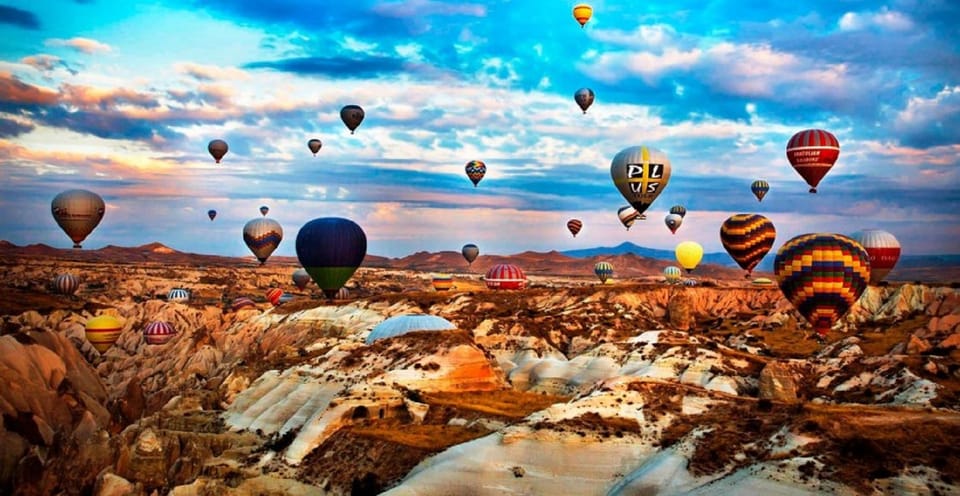The image is a panoramic view, much wider than it is tall, capturing a striking scene where numerous hot air balloons float over a rugged, almost mountainous terrain reminiscent of the western United States, possibly Arizona or New Mexico. The bottom half features a desert-like landscape with dark brownish sand, rocky hills, and valleys that transition to lighter, whitish sand areas. Dotting the horizon are black, hazy mountains. Hovering above this arid terrain, the hot air balloons vary in size and color, ranging from blue and silver to red, and some are adorned with stripes or rainbow patterns. While some balloons are tiny dots in the distance, others closer to the camera appear much larger. The top half of the image showcases a dramatic sky filled with clouds that vary from dark storm clouds to lighter ones, tinged with hues of pink and gold, suggesting either sunset or sunrise, casting a mystical light over the scene. The balloons prominently stand out against the backdrop along the skyline, adding to the picturesque quality of the image.